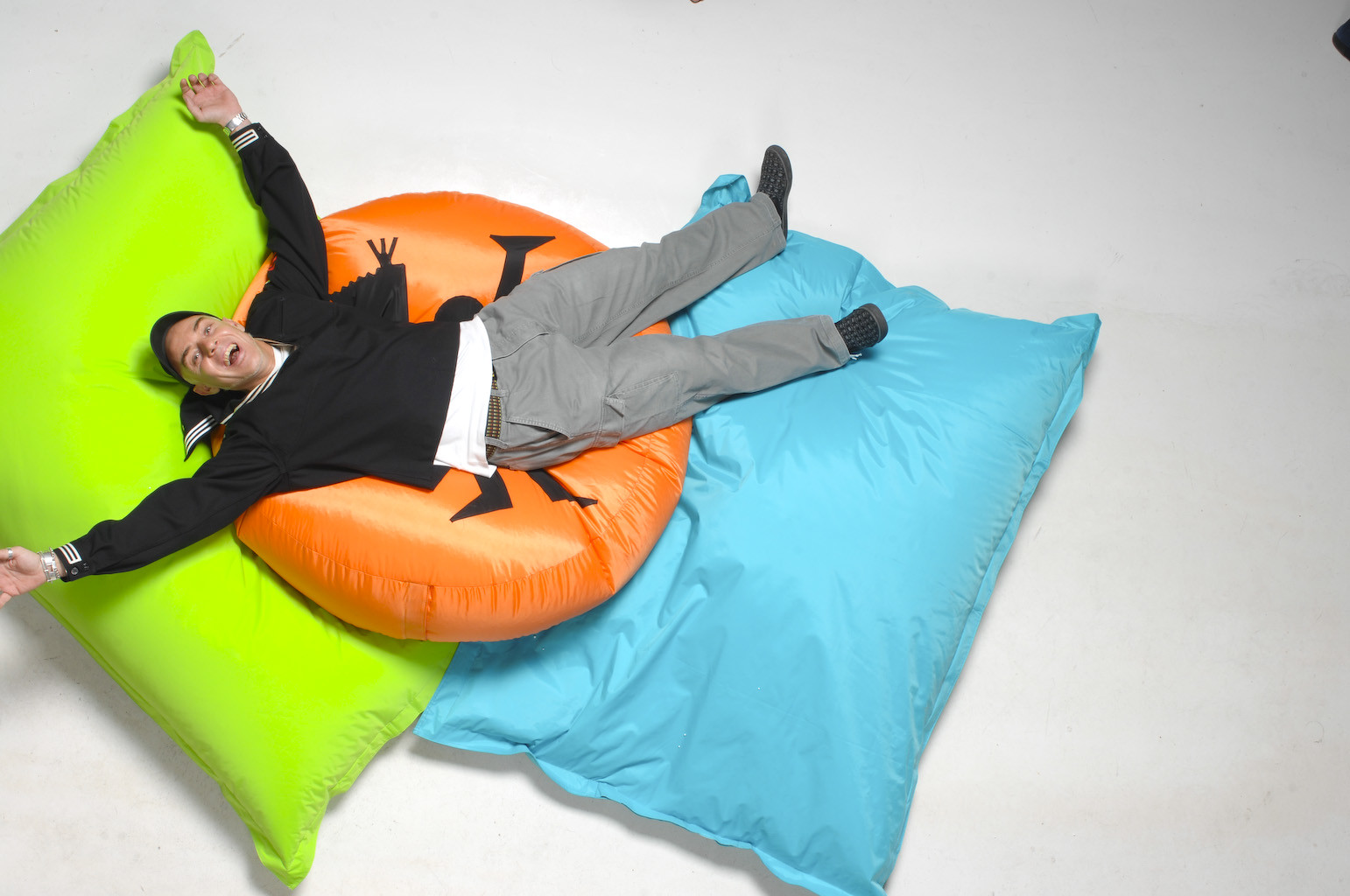In a photograph with a pure white background, a man is joyfully lounging on a playful arrangement of oversized pillows. Centered slightly to the left, three gigantic pillows form a colorful stack beneath him. At the base, there is a bright lime green, rectangular pillow, which supports a conspicuous round orange pillow in the middle, adorned with a black logo of a person. The summit is capped by a vivid sky blue rectangular pillow. The man, dressed in a long-sleeved black sailor shirt with white stripes on a broad collar, a visible white undershirt, gray pants, and black shoes with white dots, stretches out atop this stack, overlapping each cushion. With arms raised jubilantly, head tilted back, mouth wide open in a smile, and silver watches on both wrists, he epitomizes sheer delight and relaxation. His playful pose, amidst this whimsical pillow arrangement, captures a moment of unrestrained joy.